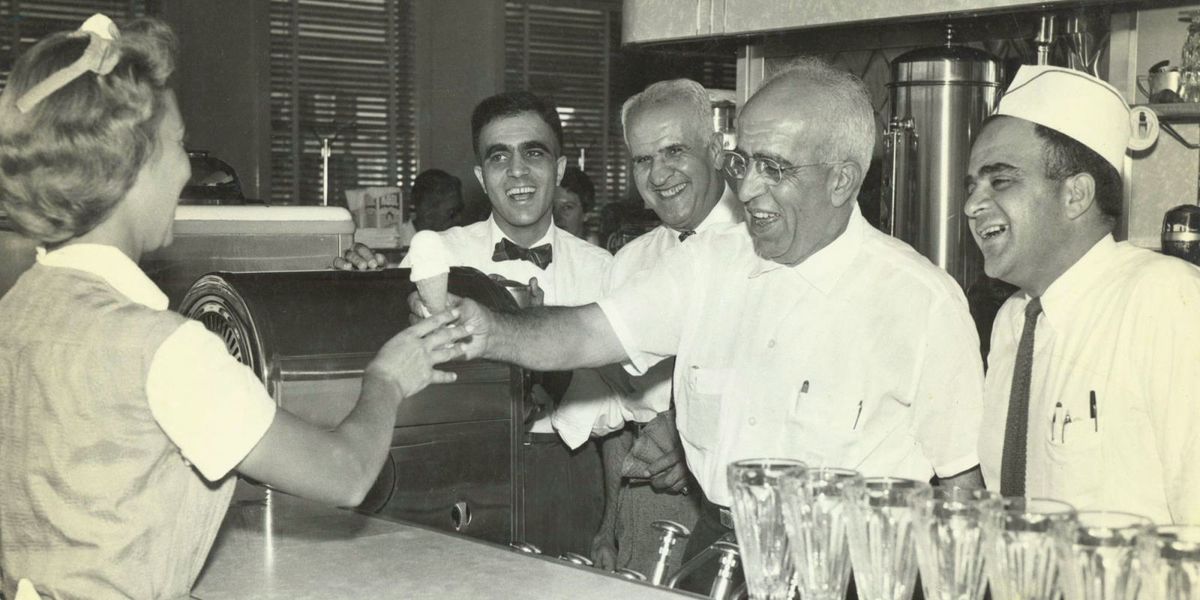This black and white photo, with a subtle yellow tint on the edges, captures a nostalgic scene inside a classic ice cream parlor or soda fountain. At the center, an elderly man with white hair and glasses, dressed in a white pocketed shirt, smiles warmly as he hands a small vanilla ice cream cone to a young waitress. She wears a sleeveless dark top over a white collared shirt, with a ribbon adorning her curly, medium-length hair. The waitress stands behind a rectangular countertop, which is adorned with a neat line of seven or eight glass sundae cups on the right. Behind the counter, there are four older gentlemen, all in white shirts. The man on the far left has black hair and a bow tie, while the younger man on the far right wears a tie and a paper hat, watching the scene unfold. Coffee machines and windows with shutters add to the charming, vintage atmosphere of the parlor.